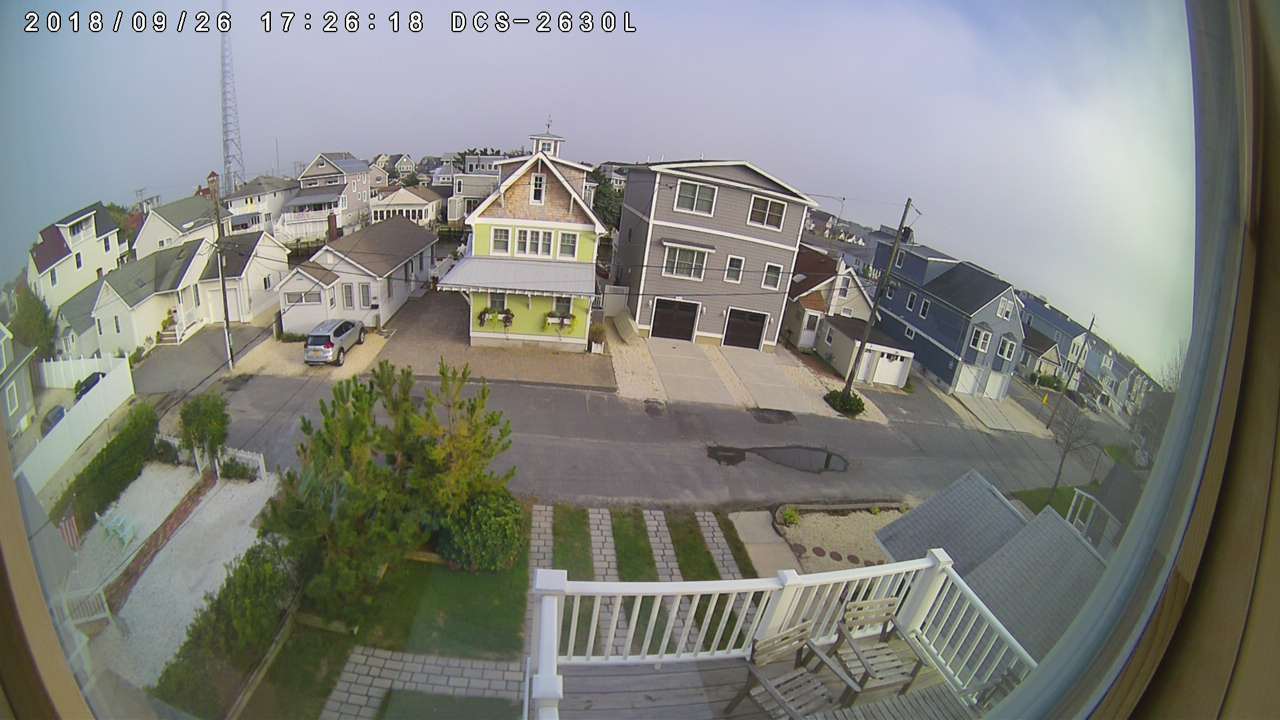The image, likely taken from a high vantage point inside a home and looking outward, captures a suburban neighborhood scene. The photograph appears to be sourced from a security camera, as evidenced by the timestamp and text "2018/09/26, 17:26:18, DCS 2630L" displayed in white font at the top left. In the foreground, there is a patio with white railing and chairs, leading to a well-maintained lawn featuring stone walkways, green grass, bushes, and a small tree with dense branches. 

The street, which may be an alleyway, runs horizontally through the center of the image, dividing two lines of houses. This street is somewhat worn and gray, with a visible pothole or puddle, and a silver car parked in front of one driveway. The neighborhood stretches into the background with dozens of houses in varying colors (yellow, dark gray, blue, and white) and heights (one to three stories). A detailed overcast sky in shades of dark blue and gray looms above. 

The image offers a panoramic-like view, showing the tops of nearby homes and featuring additional details like a large pole, possibly an electricity pole or large antenna, on the far left. The overall scene depicts a quiet suburban area with minimal activity.